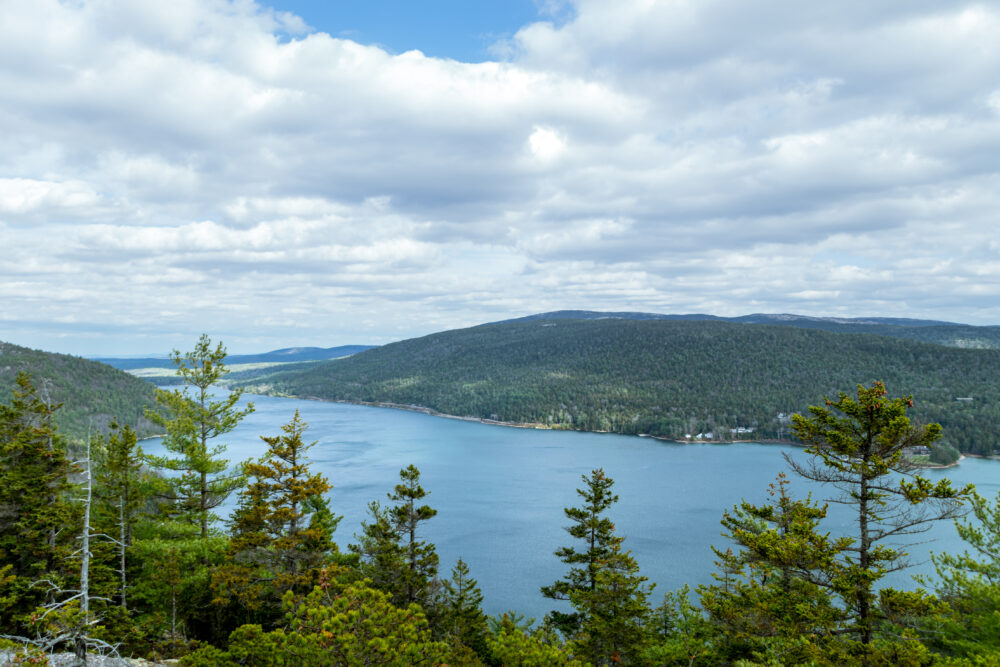This elevated landscape photograph offers a breathtaking and expansive view of a serene, turquoise-blue lake or river, surrounded by lush, verdant hills. Taken from a high vantage point—likely from atop a hill or even in the air—the image captures the sheer tranquility and clarity of the water, which stretches and meanders into the distance, suggesting that it might indeed be a river. The foreground features a dense forest of predominantly dark green pine trees, although some exhibit patches of orange and bare branches, indicating a touch of natural decay. The sky is heavily overcast with fluffy white clouds, yet fragments of bright blue manage to peek through, bringing a touch of luminosity to an otherwise cloudy day. Tiny, barely discernible structures dot the landscape across the water, highlighting the grandeur and scale of this untouched, sprawling wilderness.